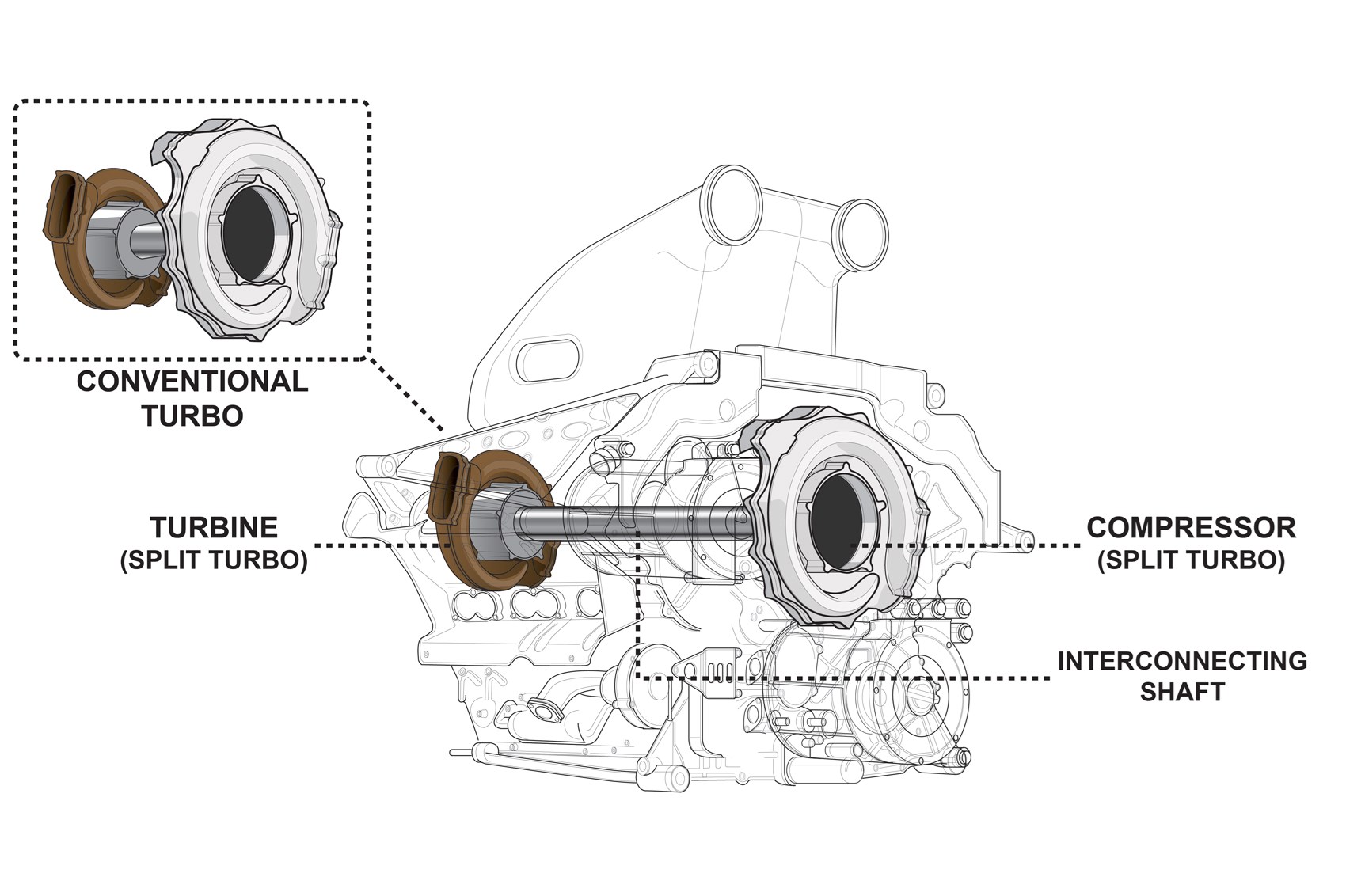This black-and-white line art technical drawing with spot color illustrates a turbine engine with a landscape orientation. The centerpiece of the image is a detailed cross-section of the engine, highlighting its inner workings. On the left-hand side, a brown ring around the crankshaft is labeled "conventional turbo" and "turbine split turbo," with a blown-up view of this section provided in a callout box above. The right-hand side features labeled callouts for the "compressor split turbo" and "interconnecting shaft," with arrows and dotted lines connecting these labels to corresponding parts of the engine. All labels and annotations are in black text, and the image is set against an infinite white background.